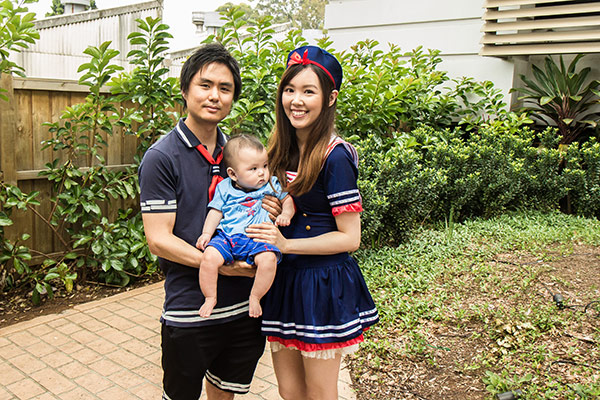In this vibrant daytime outdoor image, a young couple is the central focus as they stand slightly off-center to the left on a red brick walkway in their backyard. Dressed in modified sailor costumes, the man wears a white and blue collared shirt with a red tie and black shorts accented with white lines. The woman, adorned in a blue hat with a red bow, wears a blue outfit featuring white lines and gold buttons, likely a dress with a pleated skirt and decorative tassels. They both hold a baby dressed in a blue shirt and shorts, matching the color theme with hints of red.

The backdrop reveals a detailed residential setting. To the bottom left, the brick walkway meets a brown wooden fence that separates the yard from an adjacent property. The fence is surrounded by lush, green bushes that show hints of yellow and grow from patches of dirt. In the distant background, two houses with white exteriors and off-white or cream-colored vent areas are visible, along with some vents and chimneys. The right side frames more greenery, including a yard with green and yellow grassy patches interspersed with dirt, and a discernible black cord lying on the ground. Adjacent to the house, which occupies the top right of the image, are elements like window blinds, a railing, and possibly a deck.

This idyllic moment captures the trio warmly posed in a picturesque and well-detailed suburban backyard, emphasizing their thematic sailor attire and the detailed surroundings.